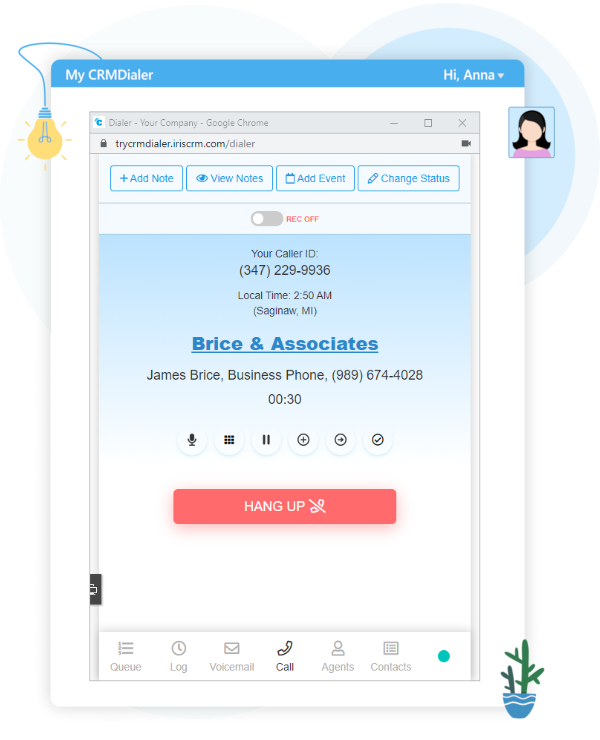**Detailed Caption:**

This image is a screenshot of an older web page. The top of the page features a blue navigation bar with the text "My CRMD Eiler" on the left-hand side and "Hi Anna" on the right-hand side next to a small icon. The icon depicts a simplistic, cartoonish face with brown hair and a pink shirt. To the left of the icon is a light bulb graphic in shades of blue and yellow.

Below the navigation bar, a line of text reads "dealer dialer your company Google Chrome try CRM dialer dot I R I S C R M dot com slash dialer." Following this, there are four rectangular blue boxes with white text inside them, labeled "Add Note," "View Notes," "Add Event," and "Change Status."

Further down the page is a section displaying information about the caller ID. The page shows the following details:

- **Your Caller ID:** 347-229-9936
- **Local Time:** 2:50 a.m.
- **Location:** Saginaw, Michigan

In larger, clickable blue text, the webpage displays "Bryce and Associates." Below this, in black text, it states:

- **James Bryce**
- **Business Phone:** 989-674-4028

A further line "00:30" follows these details, possibly indicating the duration of a call. Under this, there is a row of various icons, and at the bottom, there is a prominent red bar with white text stating "Hang Up."